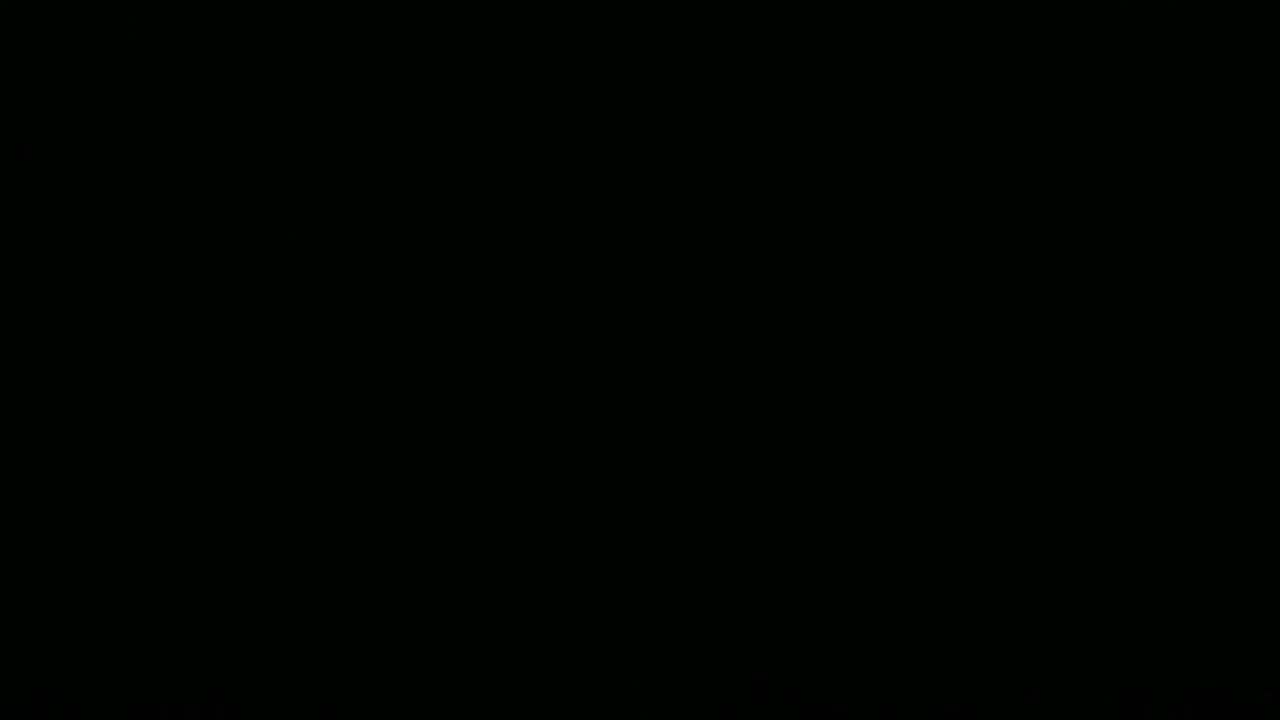This landscape-oriented image is a pitch-black rectangular box, roughly the dimensions of 12 by 8, and is devoid of any notable features. Entirely defined by its uniform, darkest black hue, there are no discernible elements such as text, gradients, or images within it. It appears as if someone captured a screenshot of a completely black background with no deviations or lightening in the shade. The blackness is consistent and absolute, much like a cleaned chalkboard or an untouched canvas, allowing no distinction between the edges and the rest of the image. This could likely serve as a setting in various contexts, such as a horror movie backdrop or a foundational element in graphic design, showcasing the versatility and timelessness of a pure black background.